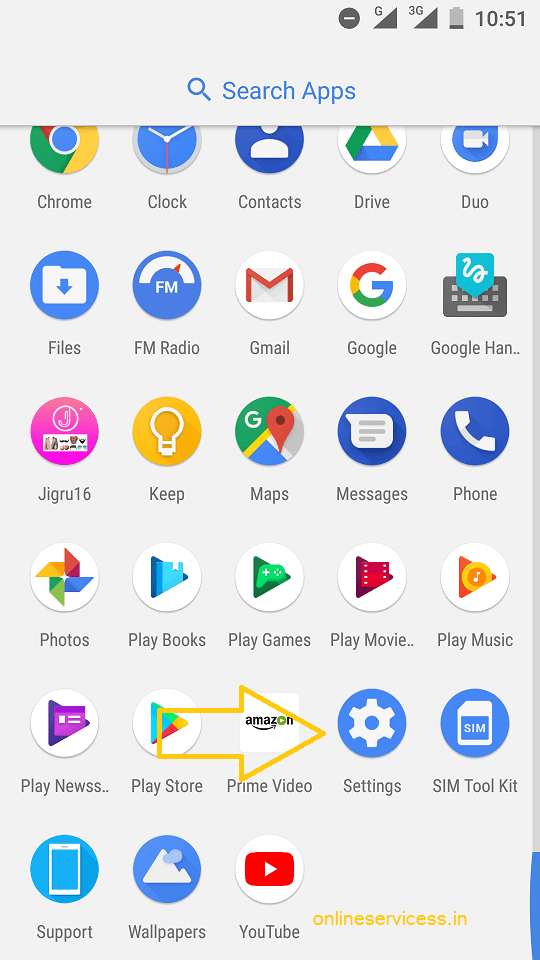The screenshot displays the home screen of a mobile device showcasing all its applications against a light gray background. At the top of the screen, there's a search icon with "Search apps" written beside it in blue. Below this, the screen is organized into six rows of app icons. Each of the first five rows contains five apps, while the sixth row has three apps, totaling to 33 apps. Starting from the top left, the first few apps are Chrome, Clock, Contacts, Drive, Duo, Files, FM Radio, and Gmail, which is characterized by a large red 'M' on a white background. This is followed by Google, G Group 16, Keep, Maps, Messages, and additional apps, completing the organized grid of icons.